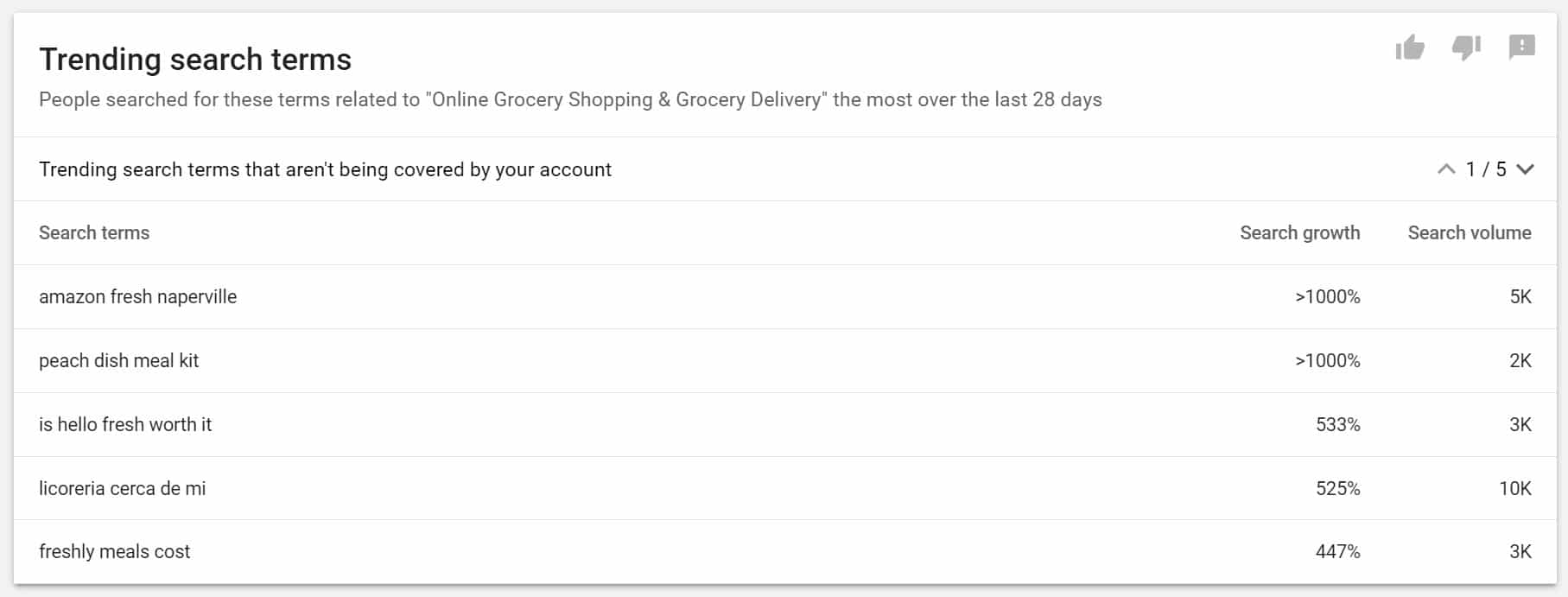This screenshot displays an analysis of trending search terms for the past 28 days, focusing on topics related to online grocery shopping and grocery delivery. The analysis reveals the top search queries that have seen the most significant increases in interest. 

At the top of the list is "Amazon Fresh Naperville," experiencing a growth of over 1,000% with a search volume of 5,000. Following closely is "Peach Dish Meal Kit," also with a growth greater than 1,000% and a search volume of 2,000. The search query "Is Hello Fresh Worth It?" has seen a 533% increase in search activity, with a volume of 3,000. "Licoreria Cerca de Mi" (translated as "Liquor Store Near Me") shows a 525% growth with a search volume of 10,000, making it the highest volume term on the list. Lastly, "Freshly Meals Cost" noted a 447% growth with a 3,000 search volume.

In the interface, there are navigation elements including 1/5 pagination indicators and pull-down/up menus. The search terms bar provides options to view search growth and search volume. In the top corner of the screenshot, there are interaction icons including a thumbs-up, thumbs-down, and an exclamation mark in a text box, allowing for user feedback on the tool’s performance.